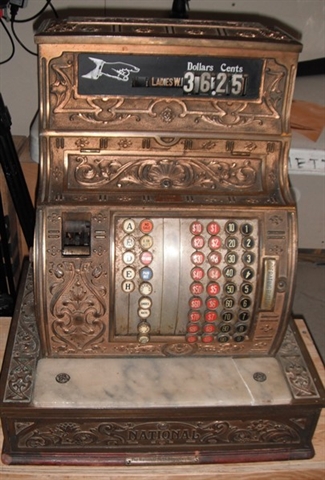This color photograph, captured in portrait orientation, depicts an antique cash register crafted from bronze-colored metal, often giving the impression of copper due to its patina. Dominating the upper portion is a rectangular black display window with "dollars" and "cents" headings, currently presenting the amounts $36.00 and $0.25. To the left within this display, a white outline illustrates a hand pointing rightward towards the price. Below this, intricate engravings adorn the brass material, reflecting the detailed craftsmanship of the era.

The centerpiece of the machine showcases multiple rows of buttons arranged to the right: two rows in red and two in black, designated for numerical inputs. To the left, there are additional rows, including one labeled with alphabetic characters (A, B, C, D, E) and another with illegible labels. Further enhancing its historical authenticity, a white marble base supports the machine, and just above the cash drawer, a conspicuous metal engraving reads "National." The cash drawer, found at the bottom of the register, shows signs of wear, suggesting extensive use over the years. The backdrop of the photograph is minimalistic, ensuring that the viewer's focus remains on the cash register itself.